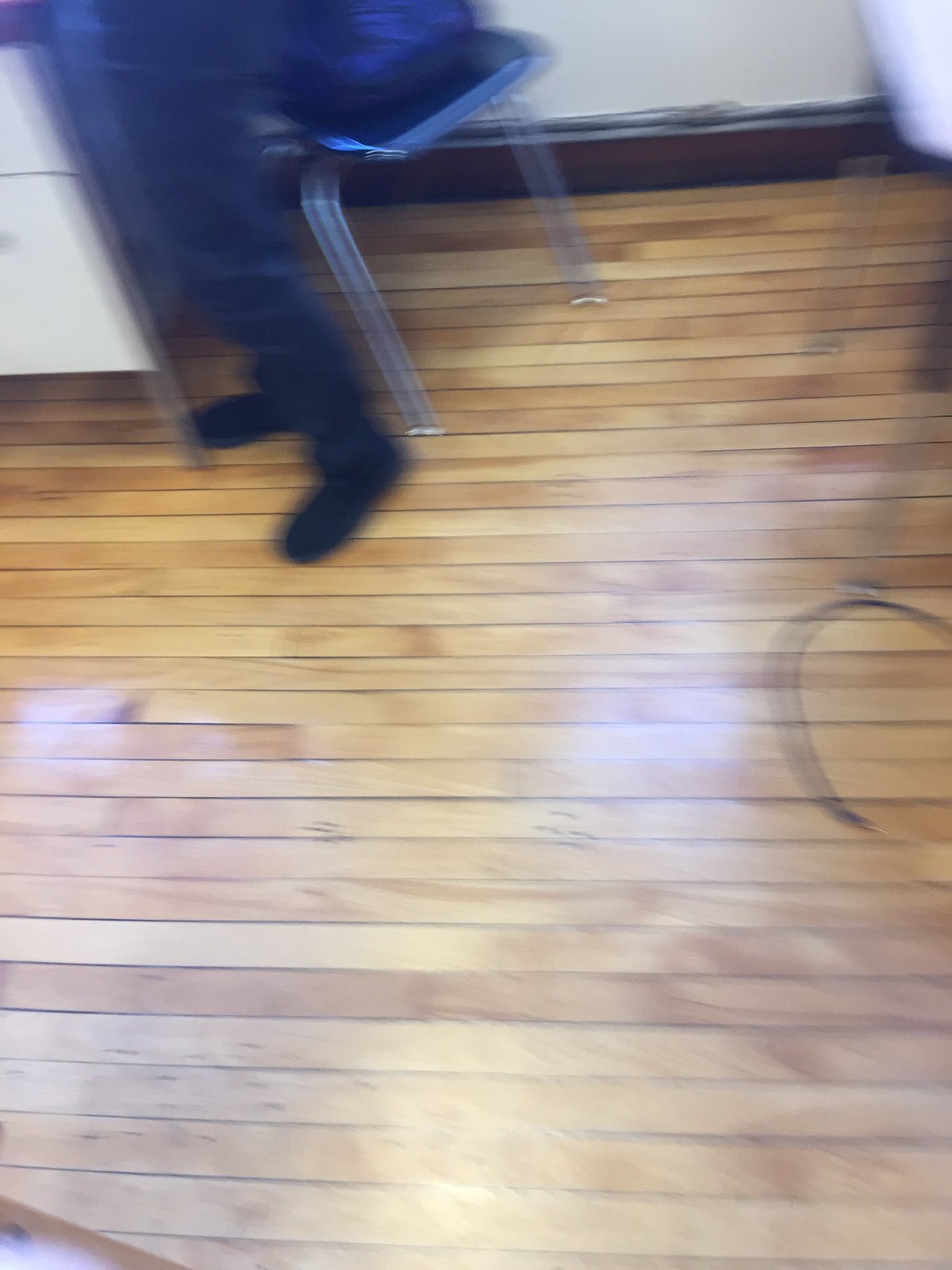This blurry indoor image depicts a scene with oak-colored wood flooring characterized by shades of yellow and brown. On the right side, a black wire snakes towards an out-of-frame destination. At the top left of the image, a person can be seen, identifiable only by their black shoes and dark pants, as they sit in a blue chair with metallic legs and a black seat. To their right, there is a glimpse of a white piece of furniture, possibly a desk with white drawers. The background features a white wall and another chair with a white seat. Additionally, there appears to be varying light patterns on the wooden floor.